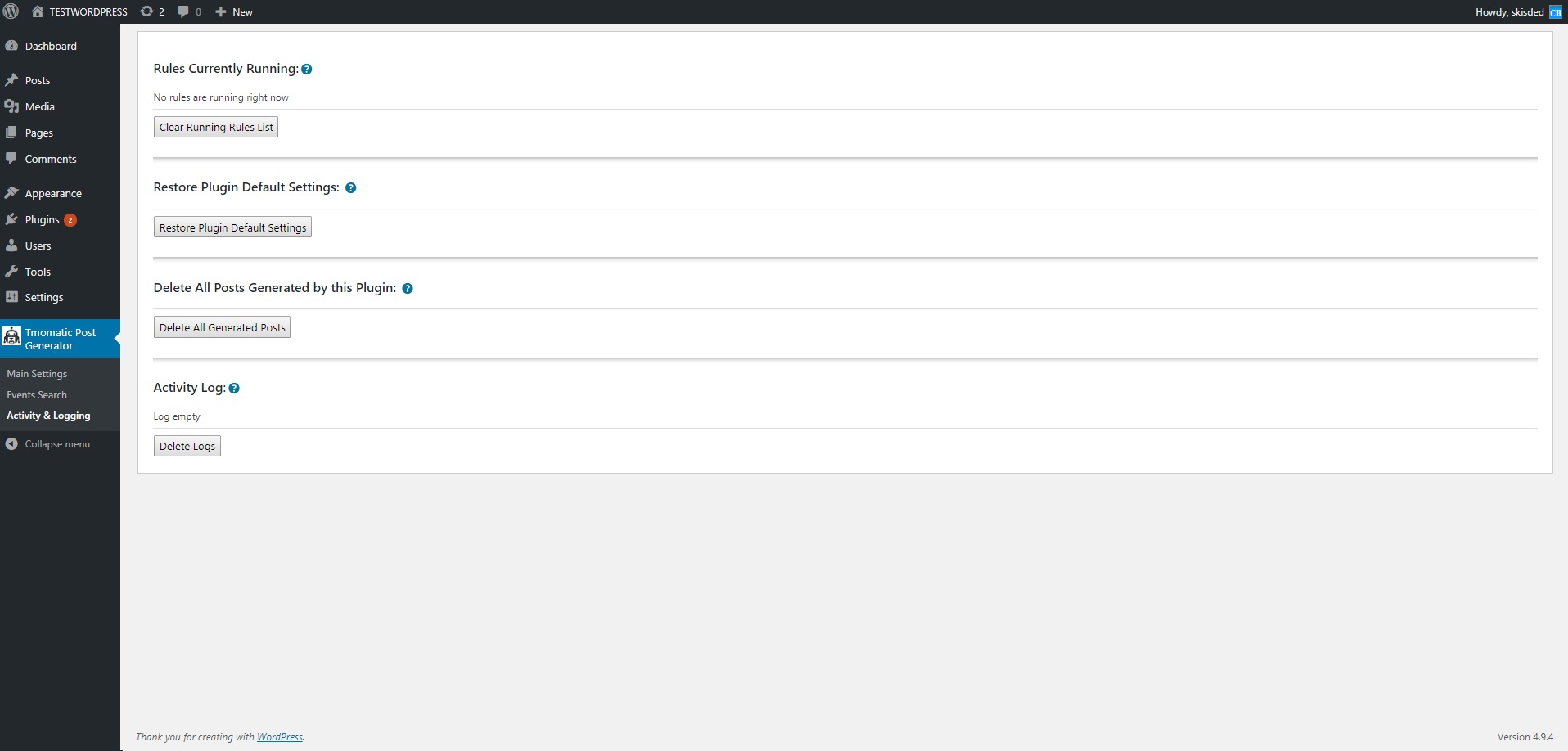This image depicts a WordPress admin dashboard with version 4.9.4 displayed in the bottom right corner. At the top left, the title "test wordpress" is visible alongside a home icon, a WordPress icon (a "W"), a refresh icon with a count of 2, a comment icon with a count of 0, and an "Add New" button marked with a plus symbol. On the top right, a greeting reads "Howdy, ski's dead."

The left side features the side menu, which contains several vertical options each accompanied by an icon. These options include Dashboard, Posts, Media, Pages, Comments, Appearance, and Plugins—the latter has a red indicator with the number 2, signifying two available plugins. Further down the menu are Users, Tools, Settings, and the highlighted "Teamomatic Post Generator" in blue. Beneath this highlighted item, the menu continues with Main Settings, Events, Search, Activity, and Login. At the bottom of the menu, there is a "Collapse Menu" option.

In the main content area, set against a white background, the top section reads "Rules currently running, no rules are running right now" with an associated button. Another section states "Restore plugin default settings" with a corresponding grey button. Further down, there's an option to "Delete all posts generated by this plugin" followed by a button labeled "Delete all generated posts." At the bottom of the content area, an "Activity log" section indicates "log empty" next to a "Delete logs" button. The page closes with a grey footer text, "Thank you for creating with WordPress," with "WordPress" highlighted in blue.